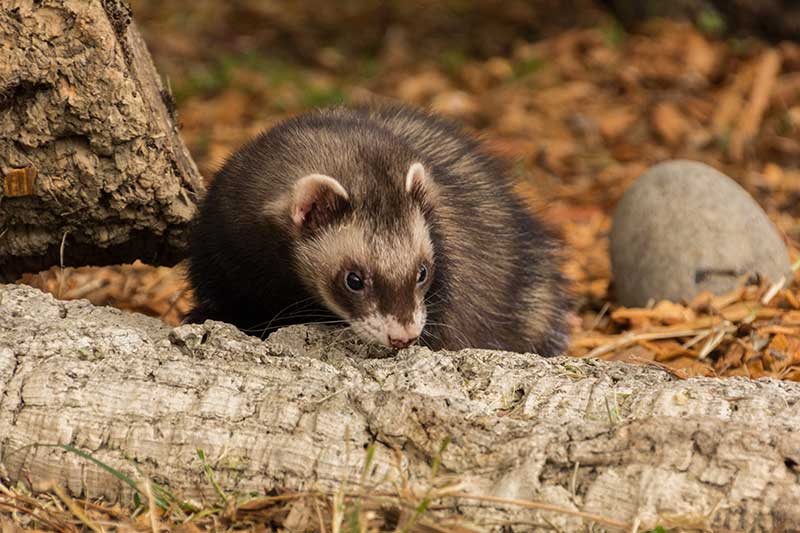This is a detailed close-up photograph taken outdoors in a natural, forest-like setting during the daytime, indicated by the bright lighting. The ground is densely covered with fallen, orange-tinted leaves and bits of tree debris, giving a strong impression of autumn. Sprinklings of green leaves add a touch of contrasting color. Dominating the foreground, there are two light-colored, almost gray logs, possibly fallen tree trunks, which run through the lower part of the image.

Centering the composition, a small furry animal, likely not a gerbil but somewhat larger, is the main subject. This unknown rodent-like creature, potentially resembling a meerkat in size and shape, features a mix of brown, beige, and white fur. Its dark, alert eyes are open and it appears to be sniffing or investigating its surroundings. The animal is positioned slightly behind one of the logs and is peeking over it, giving a sense of curiosity. A small oval-shaped stone is located to the right of the animal. The upper left corner shows a part of a tree trunk or bark adding texture to the scene. The background remains blurred, ensuring the focus stays on the detailed elements in the foreground, specifically the animal and the immediate natural surroundings. There are no other animals, people, text, or numbers present in the image.